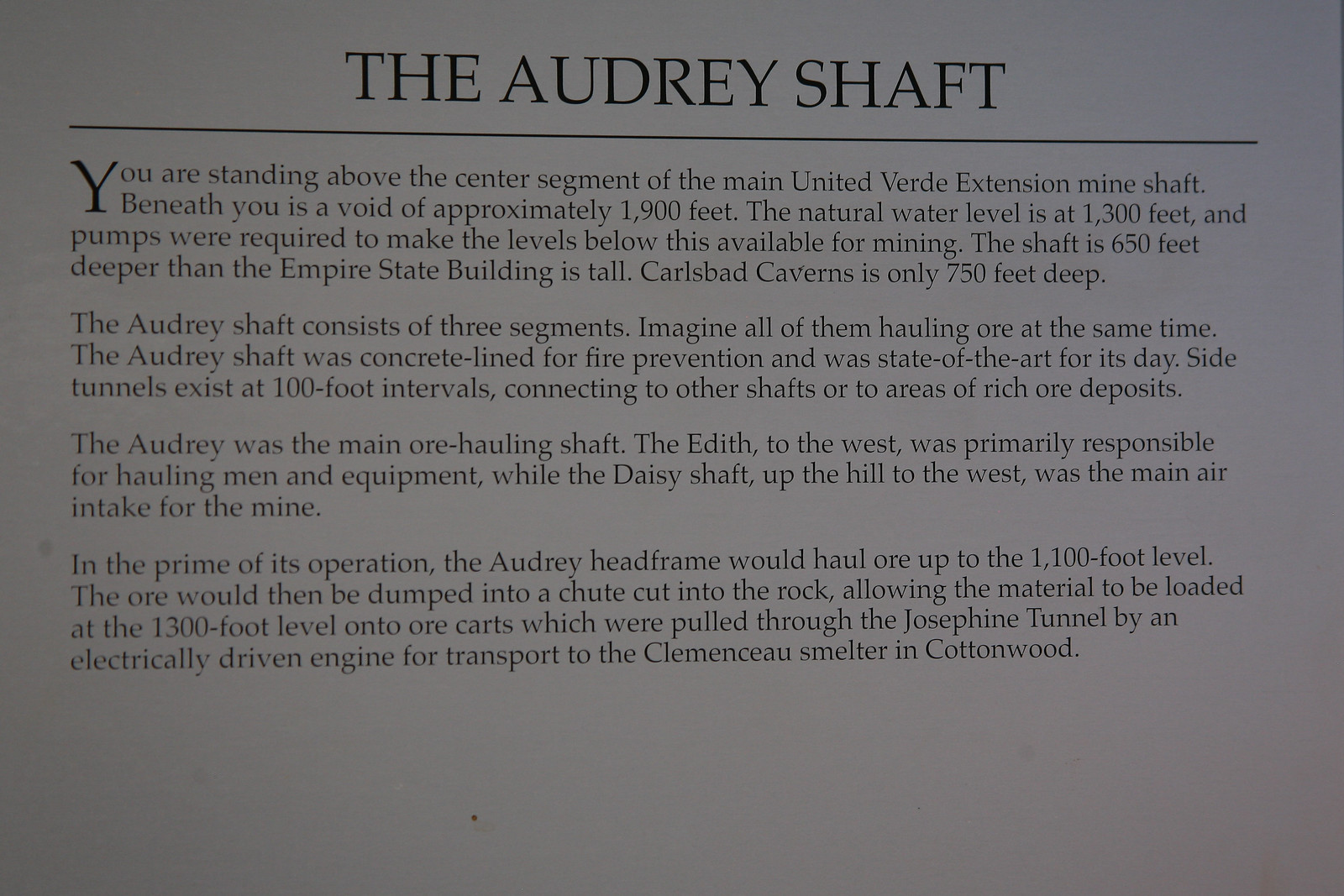This image depicts an informational placard set against a bluish-gray background, with black serif font text that is somewhat difficult to read due to poor contrast. The title, "THE AUDREY SHAFT," is prominently displayed in all capital letters at the top. Below the title, it explains that visitors are standing above the center segment of the main United Verde Extension mine shaft, which extends approximately 1,900 feet below. The natural water level within the shaft is at 1,300 feet, necessitating the use of pumps to access deeper levels for mining. Remarkably, the shaft is 650 feet deeper than the Empire State Building's height and significantly deeper than Carlsbad Caverns, which measures 750 feet.

The placard details that the Audrey Shaft consists of three segments, all operating simultaneously to haul ore. For fire prevention, it was lined with concrete, a state-of-the-art feature at the time. Side tunnels exist at 100-foot intervals, connecting to other shafts or rich ore deposits. The Audrey shaft was the main ore hauling path, whereas the Edith shaft to the west primarily transported men and equipment, and the Daisy shaft served as the main air intake. During peak operation, ore was hauled up to the 1,100-foot level by the Audrey headframe, then dumped into a rock cut chute to be loaded at the 1,300-foot level onto ore carts. These carts were pulled through the Josephine Tunnel by an electric engine to the Clemenceau Smelter in Cottonwood. The sign provides detailed historical and operational context about the Audrey mine shaft and its importance to the United Verde Extension.